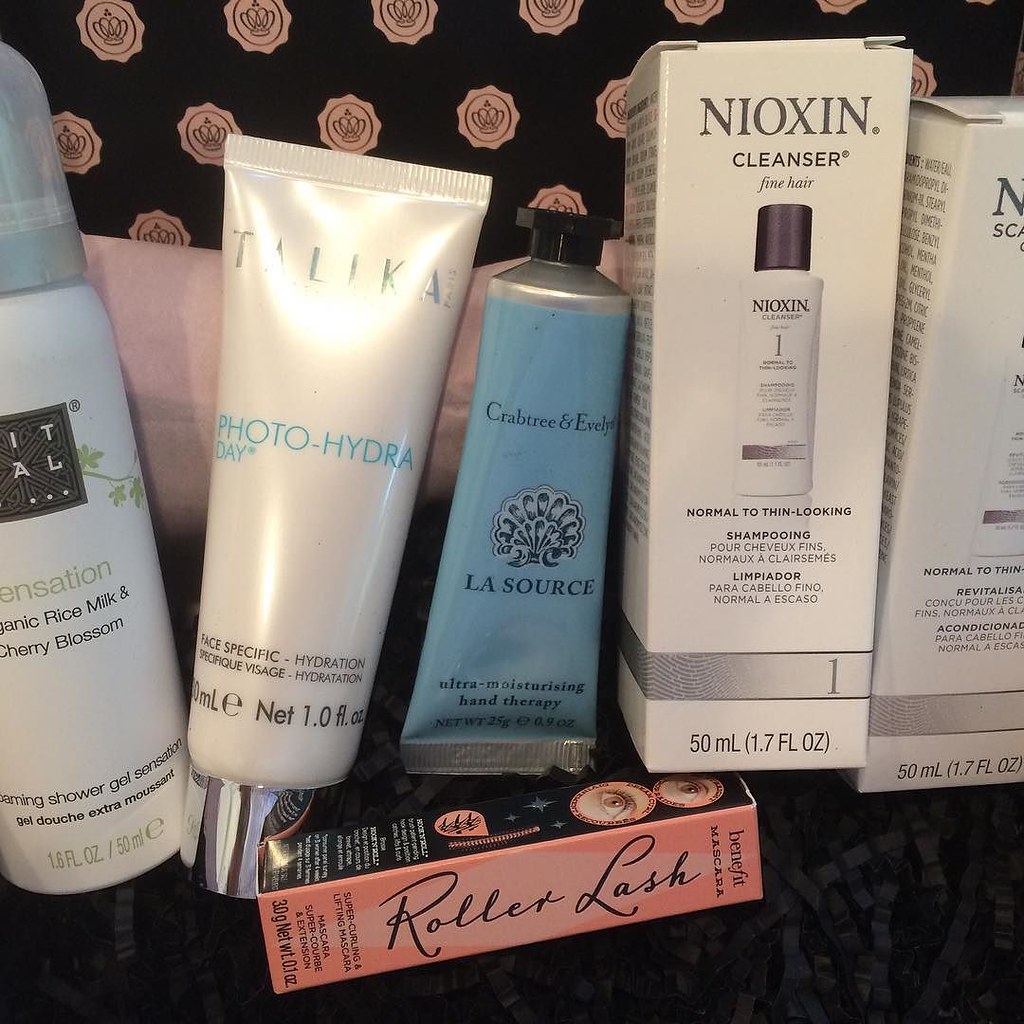The image depicts a variety of beauty products arranged in an aesthetically appealing manner against a black background adorned with pink stars. On the left side, there is a box labeled "It Owl Sensation," featuring organic rice milk and cherry blossom ingredients. Below this, there is a product called "Roller Lash" showcased in a pink box with black text and an illustration of two eyes at the top. 

Adjacent to these items is a "Talika Capture" product, accompanied by an "Evelyn La Source Ultra-Moisturizing Hand Therapy," which is a blue lotion bottle with a black cap. 

On the far right side of the arrangement, there is a box for "Neotox Neo X" facial cleanser next to another box, suggesting it belongs to a similar product line. The meticulous arrangement of these items against the striking black and pink star-patterned wall creates a visually captivating display of beauty gear.